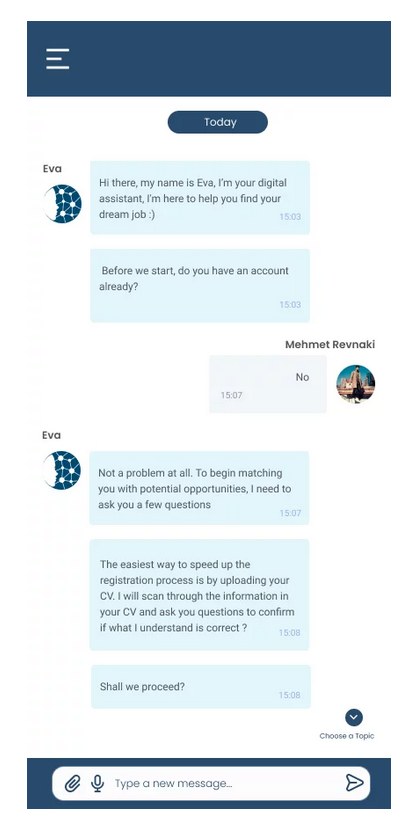The image captures a screenshot of a conversation between a user named "Mifmet Rifnaki" and an AI digital assistant named Ava. The exchange starts with Ava introducing herself and offering assistance in finding a dream job. Ava inquires if Mifmet Rifnaki already has an account, to which Mifmet responds with "no." Ava then reassures Mifmet that it's not an issue and suggests starting the process of matching with potential job opportunities. She proposes the quickest method by uploading Mifmet's CV, which she will scan to understand the user's background better. Ava plans to follow up with questions to confirm the extracted information and asks Mifmet if they are ready to proceed. The conversation effectively sets the stage for a personalized job-search experience facilitated by AI.